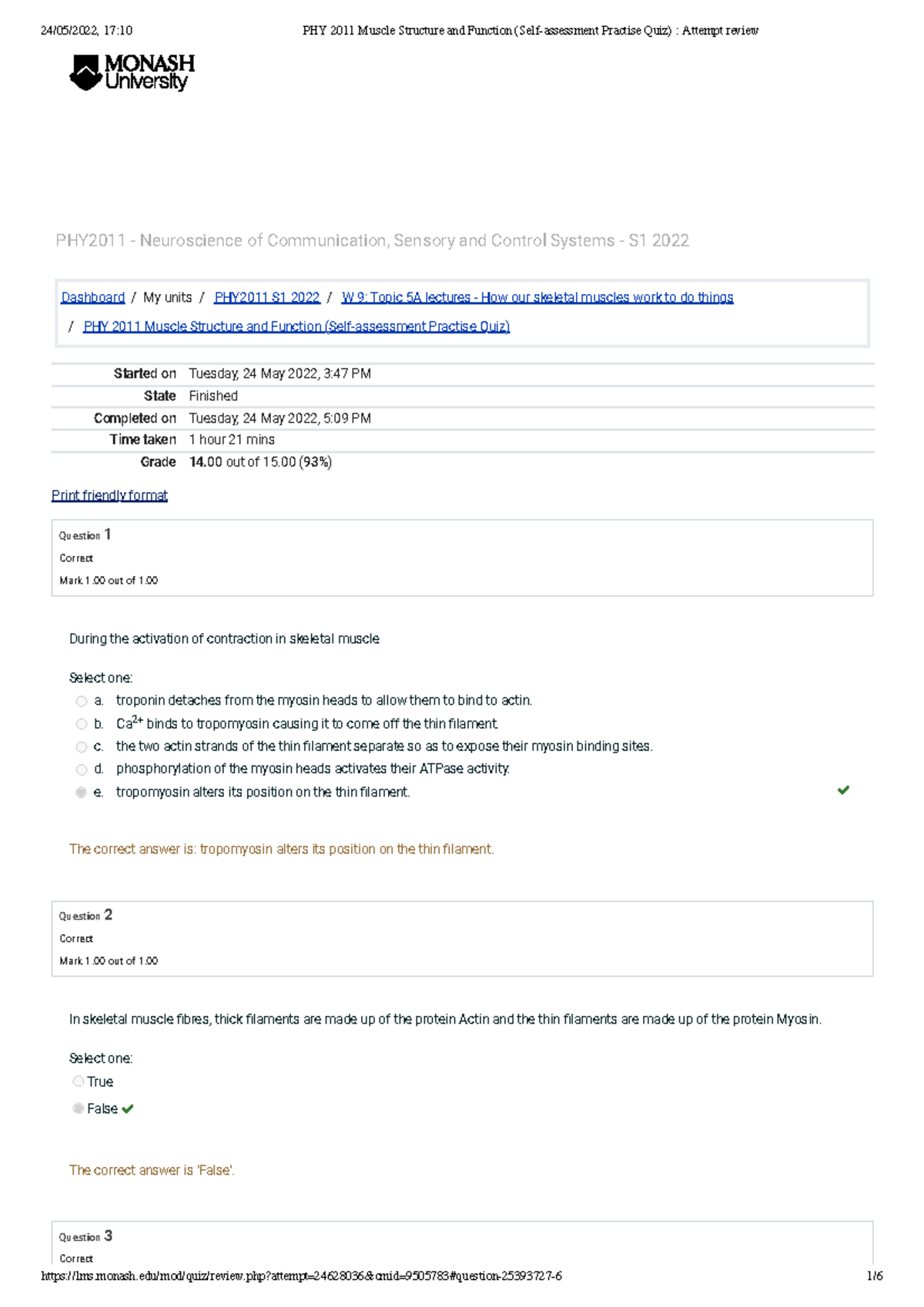The image features a clean white background. In the top left corner, the Monash University logo is prominently displayed next to a black icon. To the right of the logo, detailed course information is listed: "PHY 2011, Neuroscience of Communication, Sensory and Control Systems, S1 2022."

Below this, there is a neatly outlined box containing course navigation options such as "Dashboard" and "My Units." The box also provides specific details about a recent assessment, including its starting time on Tuesday, 24th May 2022 at 3:47 p.m., and its completion time on the same day at 5:09 p.m. It indicates that the total duration was 1 hour and 21 minutes, with a grade of 14.0 out of 15.0, or 91%, displayed in a print-friendly format.

Further down, another box appears with detailed information about the duration of activities. Specifically, it discusses the activation and contraction of skeletal muscle, where a question prompts the user to select one of five options labeled A, B, C, D, and E, each with a corresponding circle to mark the answer.

Question 2 is followed by a true-or-false question where the answer marked is "False." Additional information is provided in much smaller print toward the end of the document.